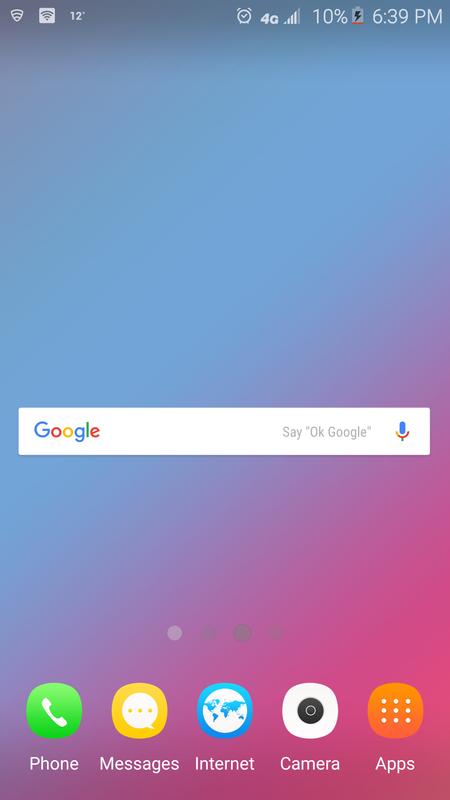Screenshot of an Android Phone Home Screen:
 
This image is a detailed screenshot captured from an Android phone at 6:39 PM. The phone's battery is critically low, at less than 10%, but it appears to be charging. The 4G network is activated, and the alarm is set, representing four out of five bars for battery indicator. The weather widget shows an outside temperature of 12°C or 12°F, although it is unclear which unit is being used.

The overall background of the home screen features a beautiful gradient that transitions diagonally from blue at the top to pink at the bottom. Dominating the center of the screen is a Google search bar, with the Google logo on the left and a microphone icon on the right next to the text "Say OK Google."

This screenshot indicates that it is the first page out of four available pages on the home screen. At the bottom of the screen, there are several app icons organized in a dock: the 'Phone' app in green, 'Messages' in yellow and white, 'Internet' represented by a globe icon in blue and white, 'Camera' in white with a black dot in the middle, and an 'Apps' button in orange.

Overall, the image provides a thorough glimpse into the user’s phone interface and its vibrant aesthetic.